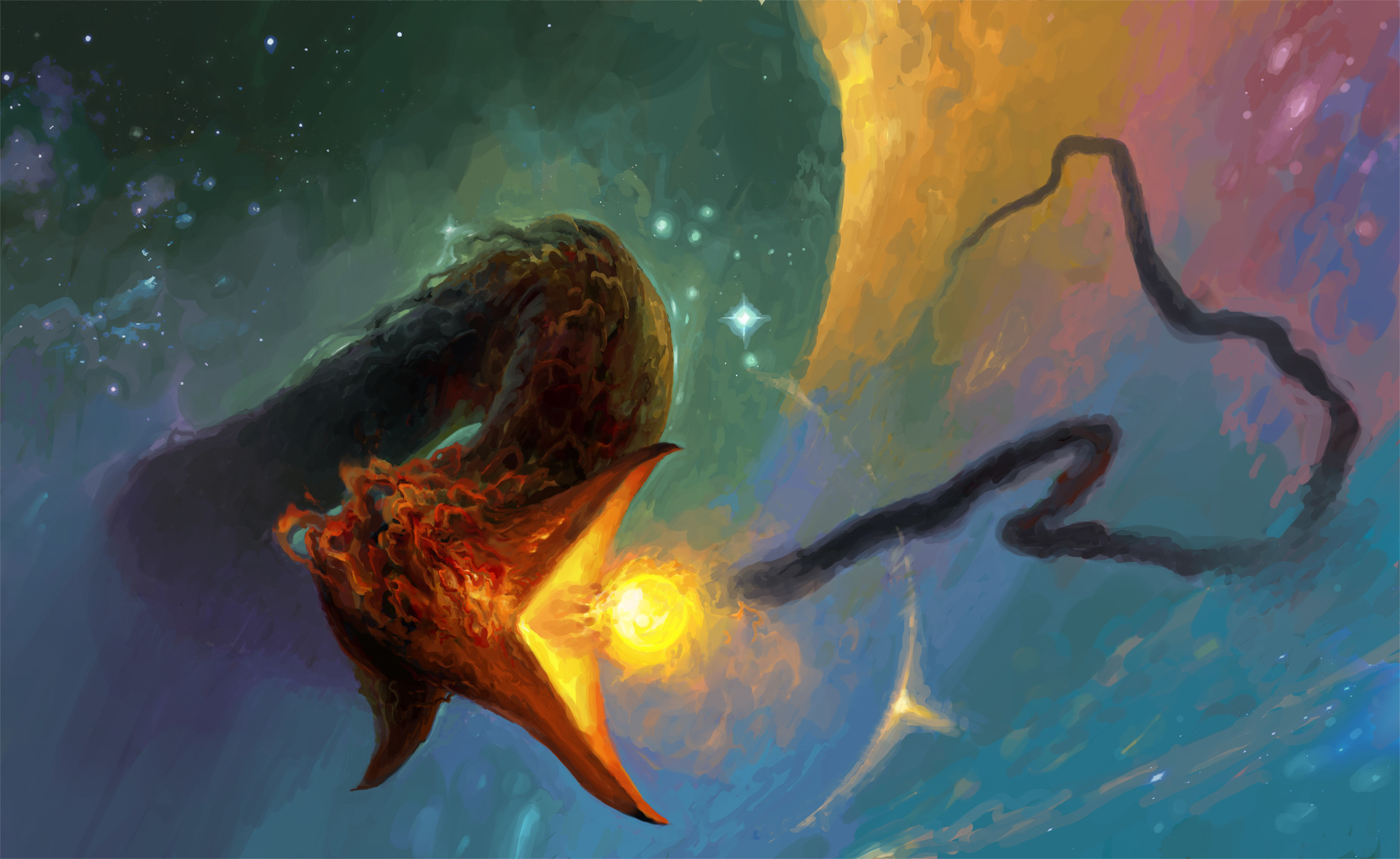This captivating piece of digital art by artist Zhengyi Wang, titled "Star Devourer," is set within a long, thin horizontal rectangle format. The artwork depicts a mythological, snake-like creature with an ominous, beak-like mouth, wide open as it attempts to consume a radiant orb of light. The creature’s elongated body meanders towards the right side of the image, juxtaposed against its menacing head located to the left. The scene unfolds in a surreal cosmic space, adorned in a delicate palette of pastel hues. The upper left corner is bathed in soft green tones, transitioning to soothing blues at the bottom. The right side of the image is a harmonious blend of yellow, pink, green, and blue, creating a visually striking contrast. The creature itself boasts a dark green, almost black body that exudes a sense of mystique, while its head is painted in a vibrant, fiery orange, accentuating its fearsome presence in the ethereal setting.